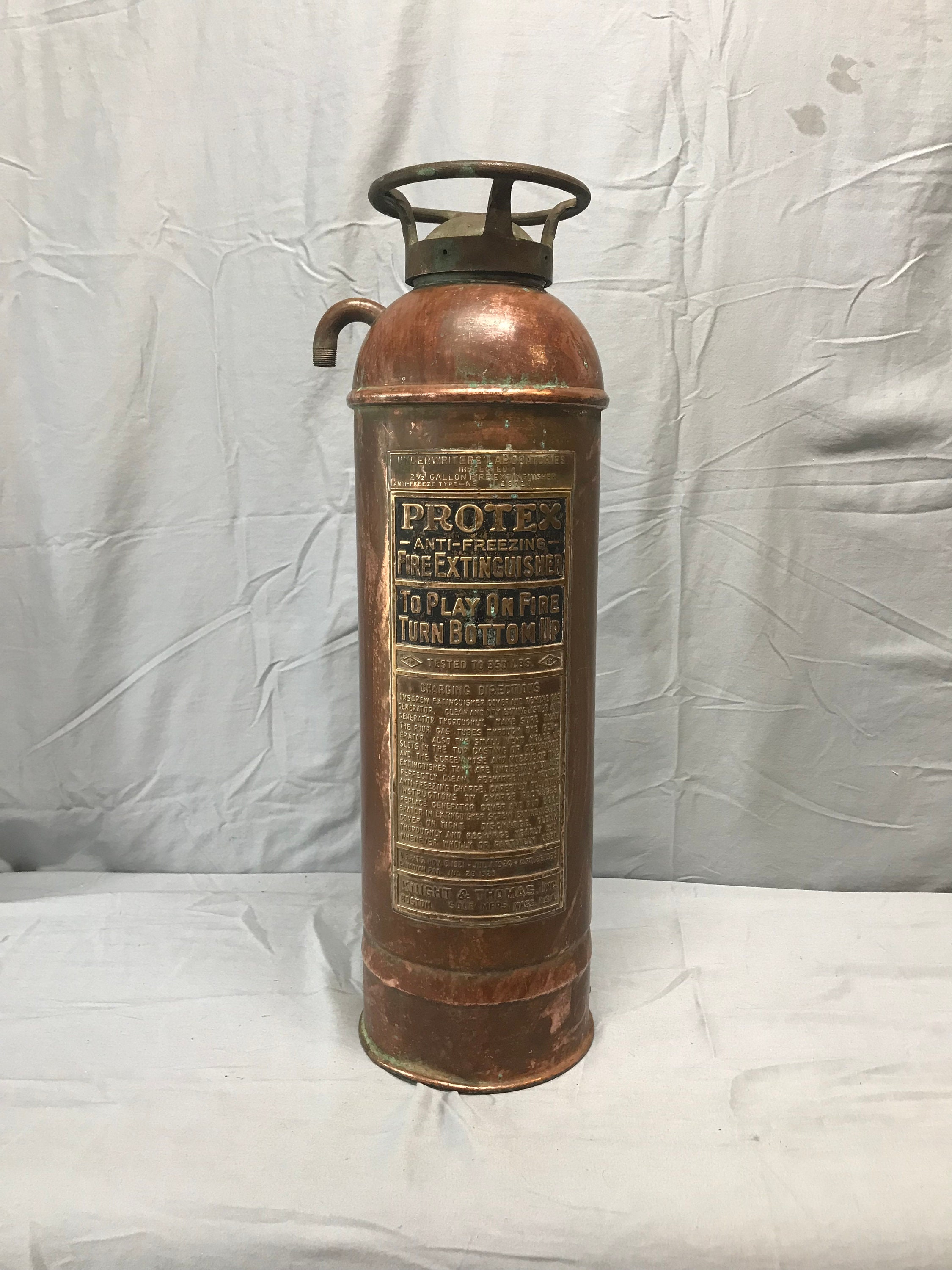This detailed photograph showcases a vintage Protex anti-freezing fire extinguisher, centrally positioned on a surface covered with a white sheet, with the background also draped in a similar fabric. The extinguisher itself has a worn, copperish-bronze appearance, indicating its age and use over the years. Notably larger than modern models, it features a turning valve at the top and a metal nozzle on the left side, suggesting sturdier, older construction methods as opposed to modern plastic components. The wording on the front, inscribed in gold, reads "Protex Anti-Freezing Fire Extinguisher. To play on fire, turn bottom up." There is additional, smaller text beneath this main label that is too fine to decipher, akin to the difficulty of reading an eye chart. The image clearly conveys the extinguisher's antiquity and historical value.